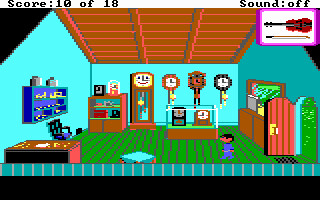This screenshot captures a scene from a vintage-style point-and-click adventure game, evoking nostalgia for retro computer games with its pixelated graphics. A character, clad in a blue jumpsuit, is seen navigating through a room that’s saturated with various timepieces. Clocks of all sizes and designs are scattered around, some prominently displayed and others encased behind glass containers, adding an element of mystery. The room itself has a distinct color scheme with a green floor and blue walls, creating a visually vibrant environment. A prominent feature in the room is a grandfather clock, standing out amongst the plethora of timekeeping devices. Above the scene, a text displays the score as "10 of 18," indicating the player's progress in the game. The overall ambiance suggests an engaging point-and-click adventure where each detail could be a crucial piece of the puzzle.